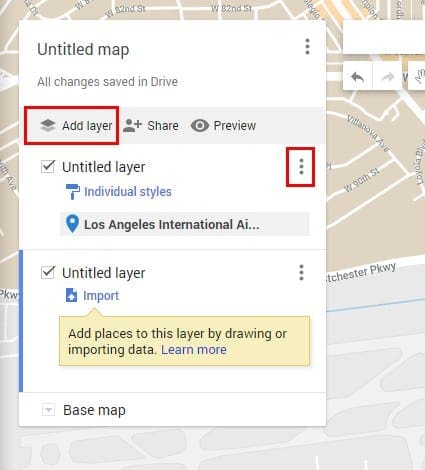The image prominently displays a central interface of a mapping application, with a background map visible. At the top of the interface, the header reads "Untitled Map," followed by a note stating "All Changes Saved in Drive." To the right, there are three vertical dots indicative of a menu.

Below the header, the interface features several labeled controls. A red box highlights the "Add Layer" button, indicating its importance. Adjacent to this, options for “Share” and “Preview” are visible. 

Further down, an "Untitled Layer" is listed with a checked box next to it, denoting its active status. Underneath, "Individual Styles" is highlighted in blue, with a pinpoint icon and the partial text "Los Angeles International AI," likely referring to Los Angeles International Airport. To the right of this layer, another set of three dots is encircled in red, similar to the "Add Layer" button.

A second "Untitled Layer" also has a checked box next to it and features the "Import" option in blue. A yellow box directs attention to "Import," accompanied by the instruction "Add Places to this Layer by Drawing or Importing Data." 

At the bottom of the interface, the term "Base Map" is displayed, presumably allowing users to select different underlying map styles or settings.